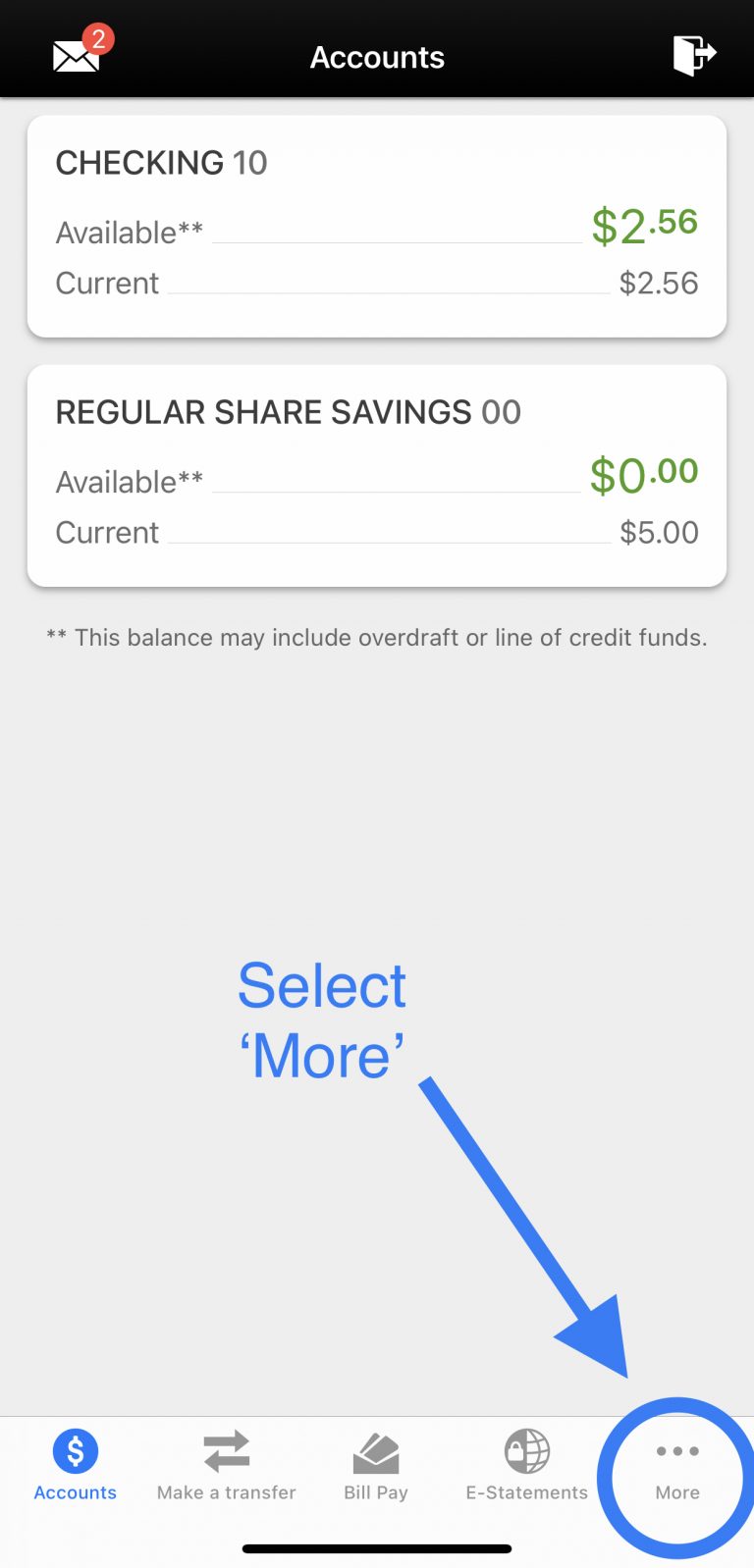The image is a screenshot of an account section within an app. At the very top, there's a black banner. On the left side of this banner, there's a small mail icon with a red circle in the top right corner, containing a white number "2," indicating two unread messages. In the center of the banner, the word "Accounts" is displayed in white text. On the right side, there's an icon resembling a door with an arrow pointing to the right, suggesting a logout or exit option.

Below the banner, the first section displays the "Checking" account information. It shows “Available: $2.56” and “Current: $2.56.” 

The section underneath provides details for the "Regular Share Savings" account, showing “Available: $0.00" and “Current: $5.00.”

A disclaimer follows, stating, "This balance may include overdraft or a line of credit funds."

At the bottom, there is a clickable option labeled "Select More," highlighted in blue, next to an arrow also pointing to the bottom right. A "More" button, circled and highlighted in the same blue, is visible.